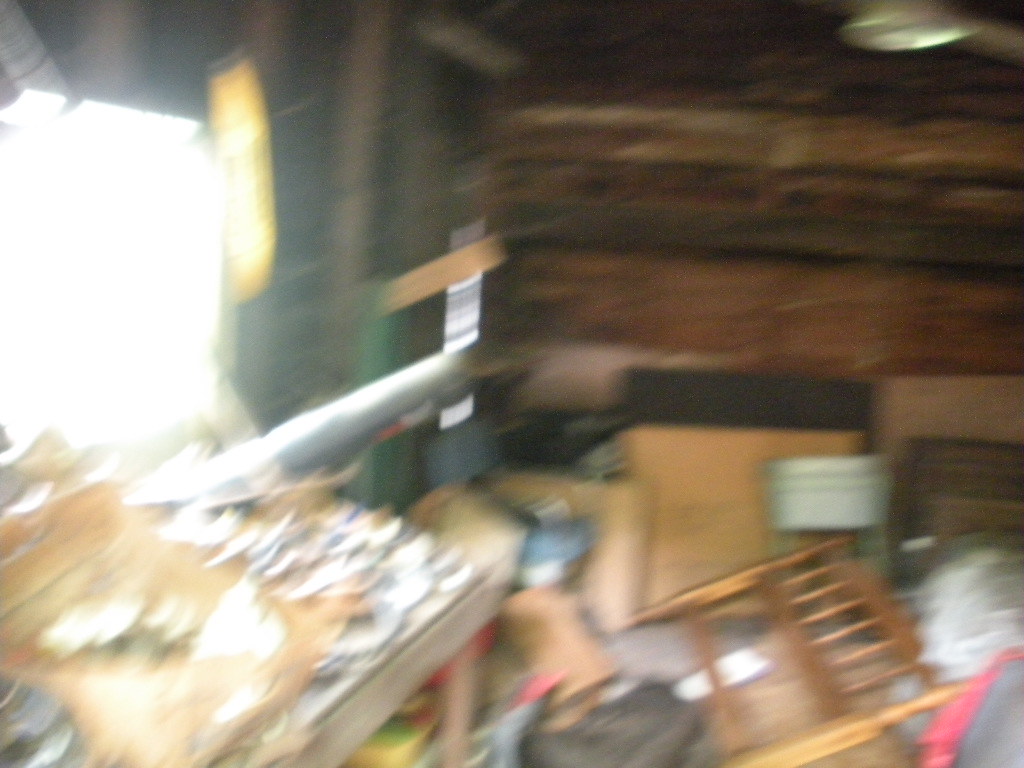This photograph, taken inside a cluttered storage area or shed, is extremely blurry but reveals a chaotic scene of disarray. The walls appear to be rough, made of wooden boards or logs. On the left side of the image, there's a distinctly bright light streaming through what could be a window or mirror, casting a glare that makes details difficult to discern. Directly in front of this light source is a wooden table almost completely obscured by a variety of objects and debris, including what appear to be papers, plates, and possibly cardboard. To the right upper corner, a large brown area suggests the presence of wooden furniture, possibly part of a larger structure. In the bottom right corner, there's an unmade bed frame with wooden legs and slats, alongside a plethora of items including a leaning child’s crib, a table lamp, bags of trash, and what might be cardboard boxes and a backpack, emphasizing the room's overall state of chaos and neglect.